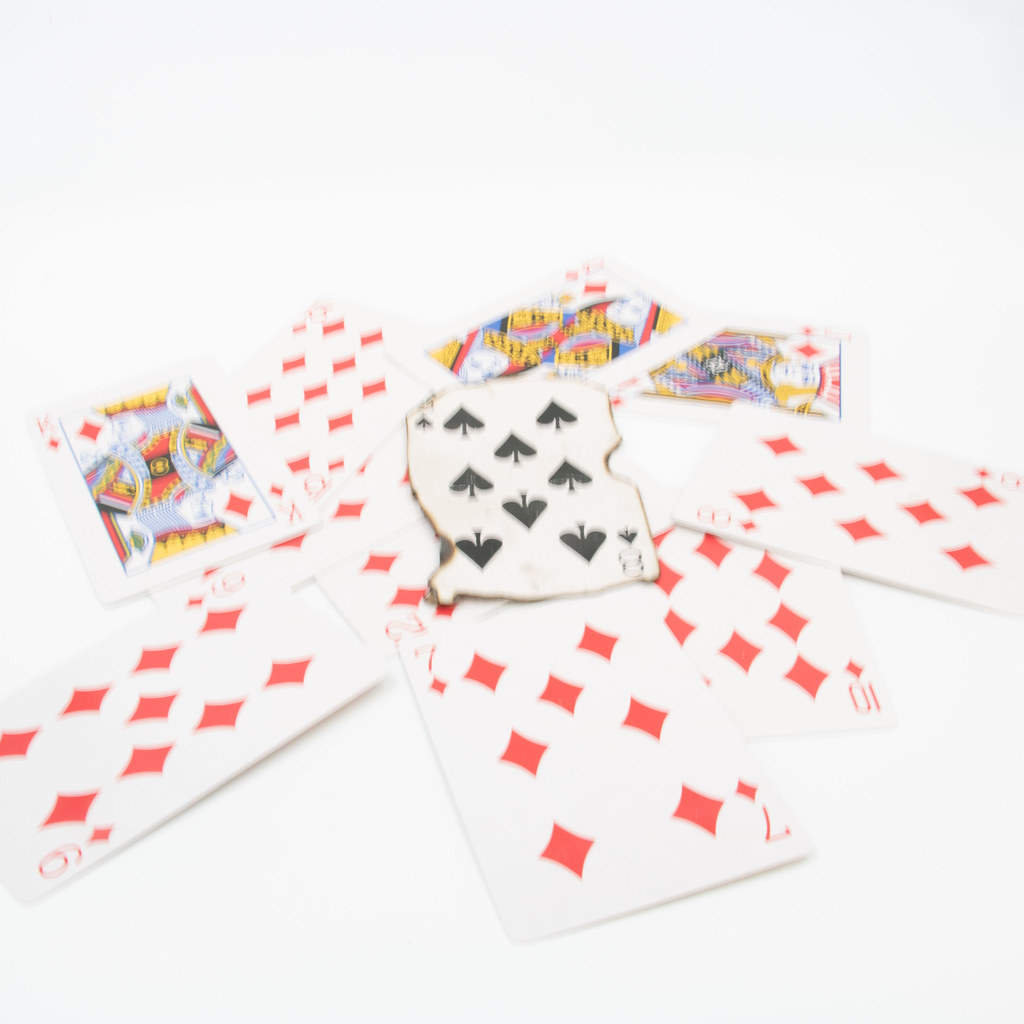This image is a color illustration rendered from a photograph, likely manipulated using Photoshop to achieve a distinctive artistic effect. The saturation is deliberately low, with the primary colors being white, red, black, and hints of yellow. It's an intricate composition of playing cards from a deck, specifically the suit of diamonds. The cards are arranged in a fan pattern, showcasing the eight of diamonds, the ten of diamonds, the seven of diamonds, the nine of diamonds, the two of diamonds, the six of diamonds, and the king of diamonds. 

At the center of the fan lies the eight of spades, which stands out due to its burned, singed edges that give it a darker and more dramatic appearance. The background features additional diamond cards, suggesting the presence of the jack, queen, and king from other suits. These face cards are depicted in a traditional style, each one mirrored so that both the top and bottom halves reflect a king, queen, or jack. This layout ensures that the cards are easily recognizable from either direction. Overall, the illustration blends intricate detail with a stylized, subdued color palette to create a visually captivating and unique representation of playing cards.